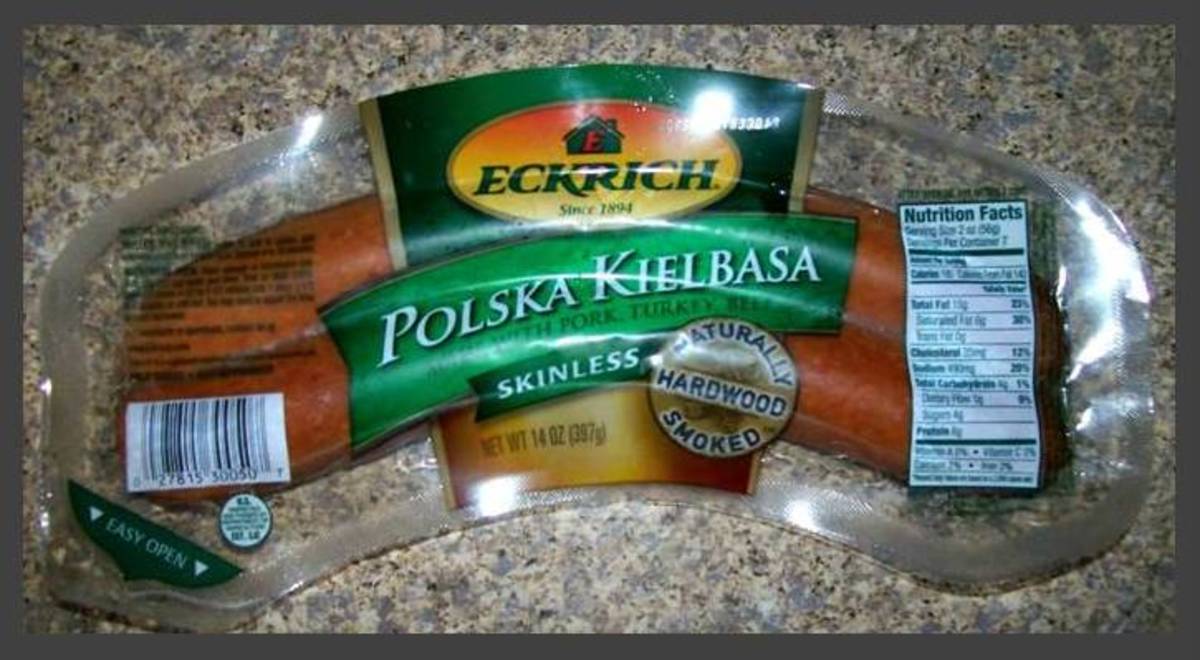This photograph, taken in a kitchen, captures a single food product – Polska Kielbasa sausage – prominently positioned in the center of the image. The sausage is encased in its original clear plastic packaging and rests on a multi-colored, smooth-textured countertop. The background features a vibrant array of colors including green, red, orange, various shades of brown, tan, gray, yellow, and other hues. Encapsulating this scene is a dark gray frame.

The packaging proudly displays the food brand, "Ekrich, since 1894," with the colors green and bronze being most noticeable on the label. Text on the package highlights that the sausage is made from pork, turkey, and beef, and is skinless and naturally hardwood smoked. Additional details include a nutrition facts section on the right side of the packaging, a barcode on the bottom left, and an easy-open green tab on the left side. The label also mentions the net weight of the product as 14 oz (397 g). The comprehensive and detailed descriptions of the ingredients are inscribed above the barcode.